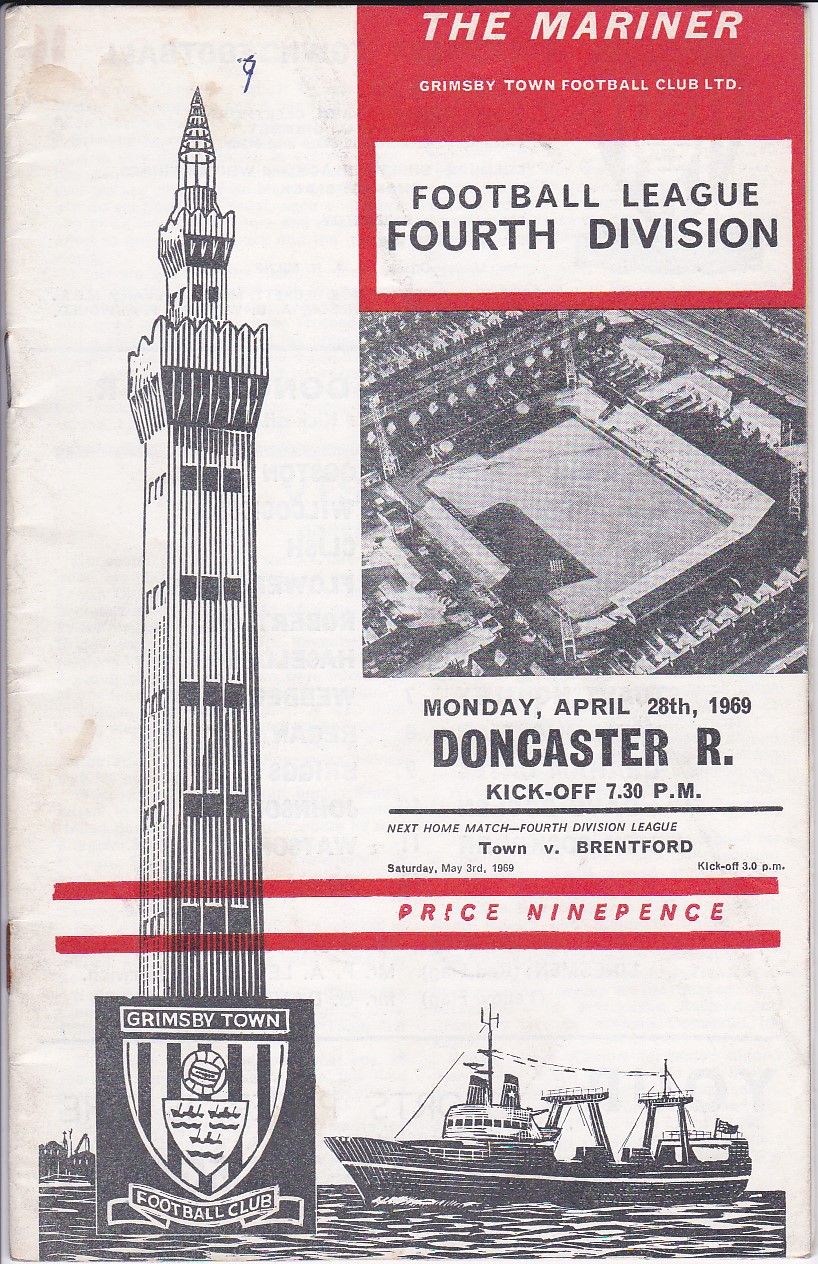This black and white 1969 football program cover for Grimsby Town Football Club features a distinctive red hue accentuating certain elements. At the top right corner, "The Mariner" is prominently displayed in red, followed by the club’s name in both white and black text, stating, "Grimsby Town Football Club Ltd" and "Football League, 4th Division." Below this, an aerial black-and-white illustration of their stadium captures an empty field. Beneath the stadium illustration, the details of an upcoming match are listed: "Monday, April 28, 1969, Doncaster R, kickoff 7:30 PM." Additionally, a small notice announces a future match: “Next Home Match, Fourth Division League, Town v Brentford – Saturday, May 3rd, 1959, kickoff 3 PM.”

To the left side, a historical and symbolic imagery is presented with an old fishing boat sailing on water alongside a detailed drawing of a tall lighthouse. Below these images, a medal-like emblem featuring a shield with a soccer ball and ribbon is inscribed with "Grimsby Town Football Club." At the bottom, framed by thin red bars, the entry price is clearly visible: “Price, nine pence.” This program cover blends maritime elements with football heritage, capturing the essence of Grimsby Town Football Club.